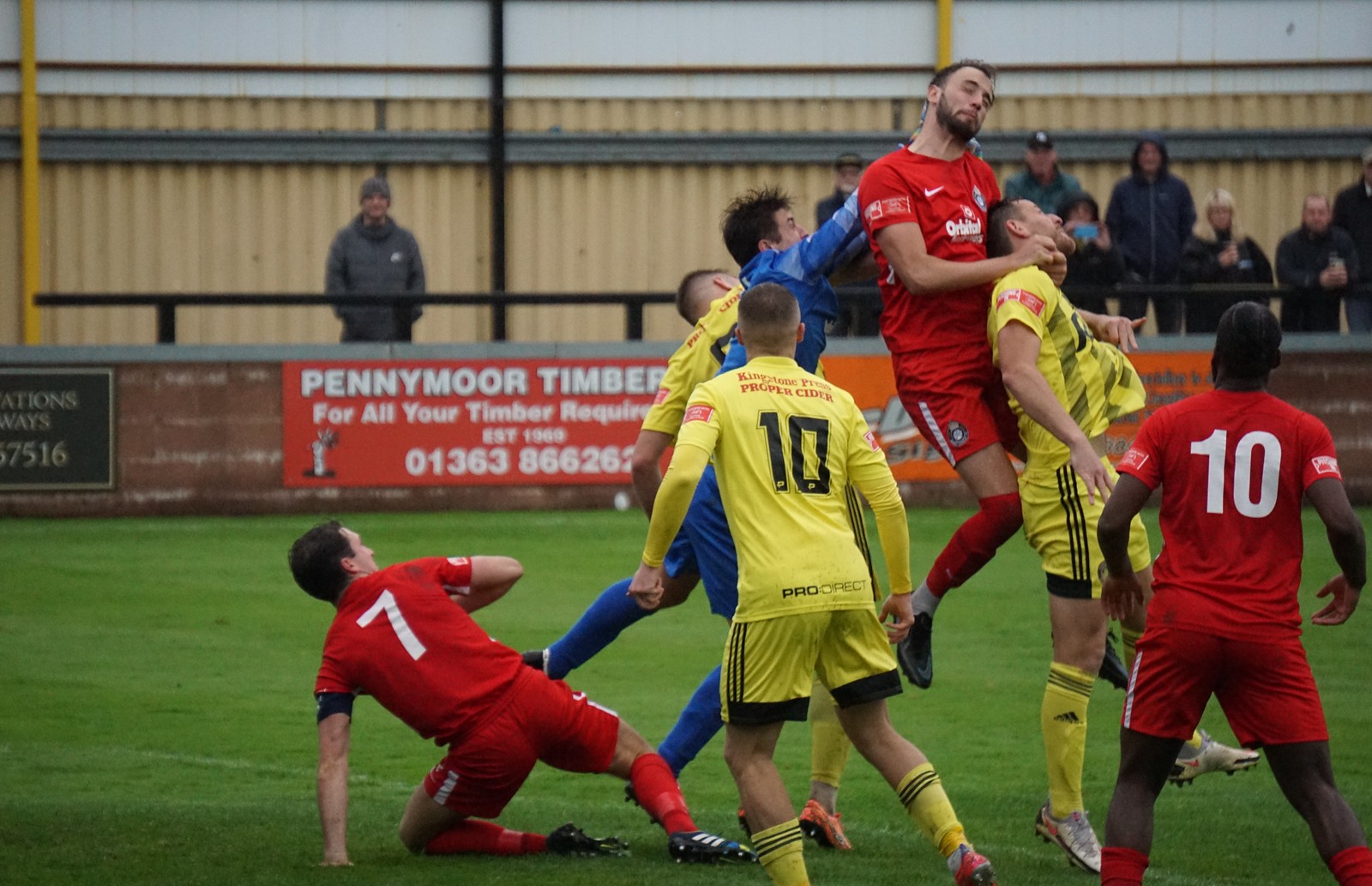In this dynamic daytime outdoor soccer match, players from two teams, one clad in red uniforms and the other in yellow, are engaged in a heated moment on a grassy field. The background features a cream-colored steel wall with banners, including one red banner from "Penny Moore Timber" advertising timber services. Behind a half-wall fence, spectators are watching the intense action unfold. 

The focal point of the image shows seven men; on the left, a player in red shorts and a red t-shirt with the number 7 and short dark hair stands next to a Caucasian player in a yellow uniform, with a shaved head. On the right edge, another player, African American, wears a red uniform with the number 10. Directly in front of him, a yellow-clad player appears to be in a chokehold by a jumping player in red with short dark hair and a beard. Behind this struggle, a man in blue, potentially the goalkeeper, is seen intervening, either holding up or pulling apart the players, though his actions are partially obscured by those in yellow and red.